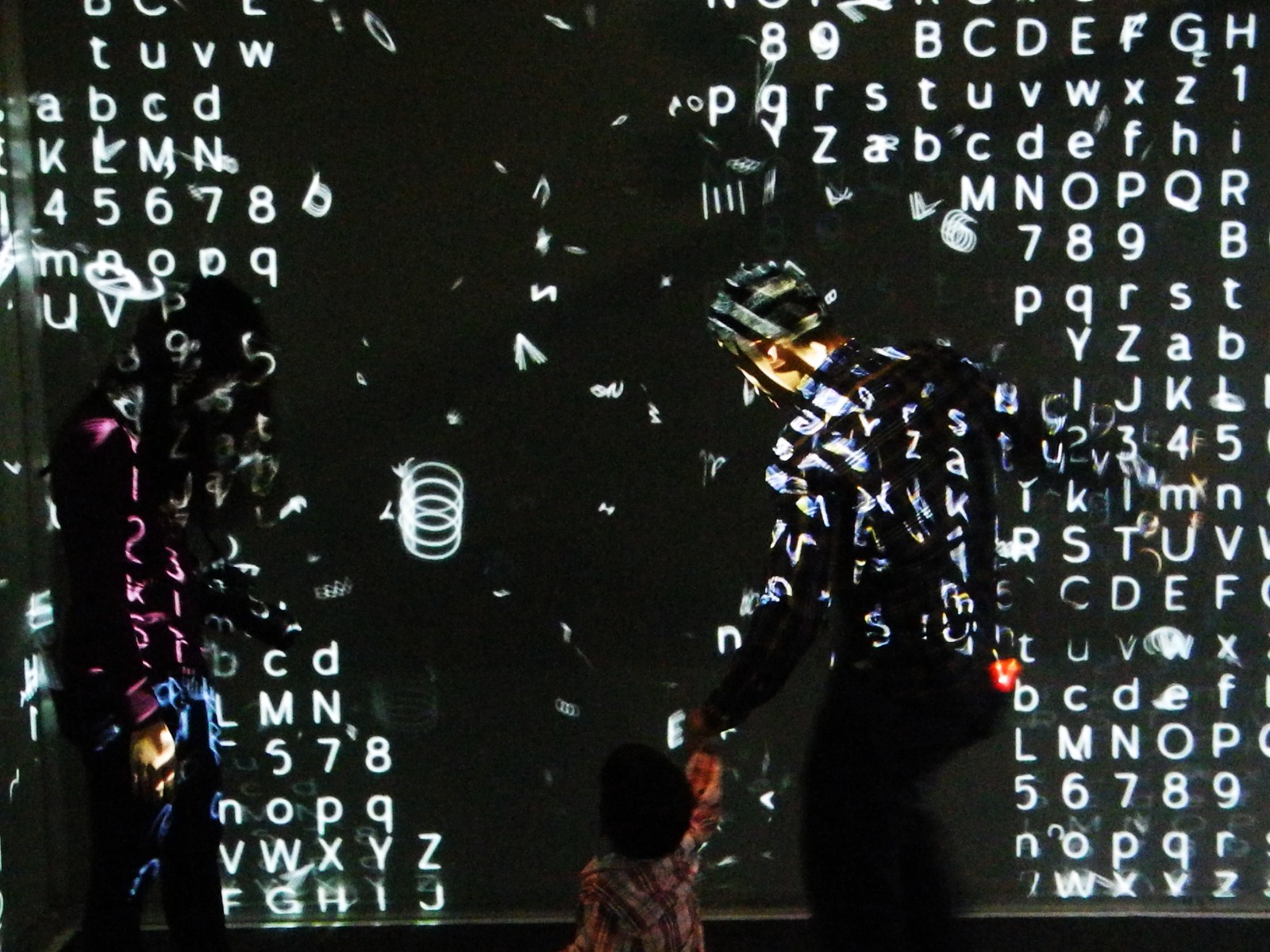The image features a futuristic design with a young man on stage, dressed in black clothing. His face is somewhat obscured as he appears to be bending down, possibly interacting with another figure in a checked shirt. Surrounding the man, on both the left and right sides of the image, are scattered letters and numbers. These characters are in various colors, including white, pink, and blue, some of which are uppercase and lowercase, with a peculiar emphasis on the letter 'N.' The arrangement of these characters appears random and abstract, lacking a discernible order. Additionally, parts of the man's clothing bear similar letters and numbers, adding to the overall avant-garde aesthetic of the design. Despite the chaotic overlay of text, the scene portrays a sense of calm and confidence emanating from the individual, suggesting that he is unfazed by the complexity around him.